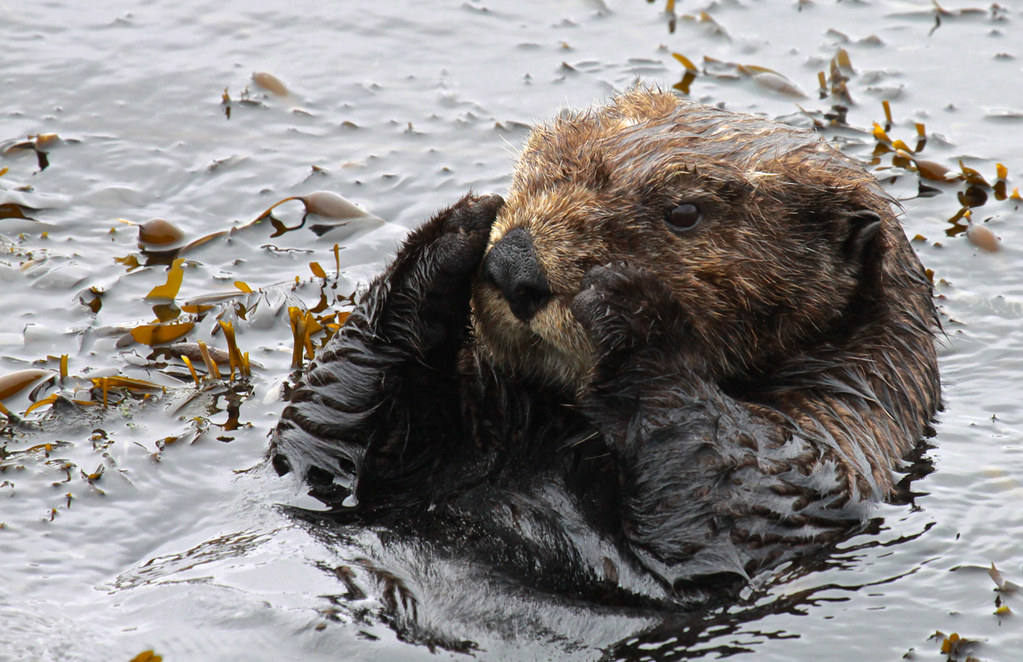The photograph depicts an adorably detailed scene of an otter floating leisurely on its back in a kelp bed. The image, captured in high-quality color under the bright daylight, exhibits the otter's rich brown fur, which appears almost black in wet areas where it clumps together. The otter's head is mostly dry, with the tips of its fur slightly wet, giving it a brushed-back look. Its black nose and dark brown eyes are prominently visible as it gazes directly at the camera. The otter's paws are adorably placed on either side of its snout, contributing to its cute, endearing expression. The water surrounding the otter is a mixture of crystal-clear and grayish hues, suggestive of a cloudy sky reflection. Floating around the otter are dark green kelp leaves, adding a natural touch to the serene aquatic setting. The clarity and vividness of the image highlight the detailed textures of the otter's fur and the surrounding environment, making the photograph an exquisite capture of nature's charm.